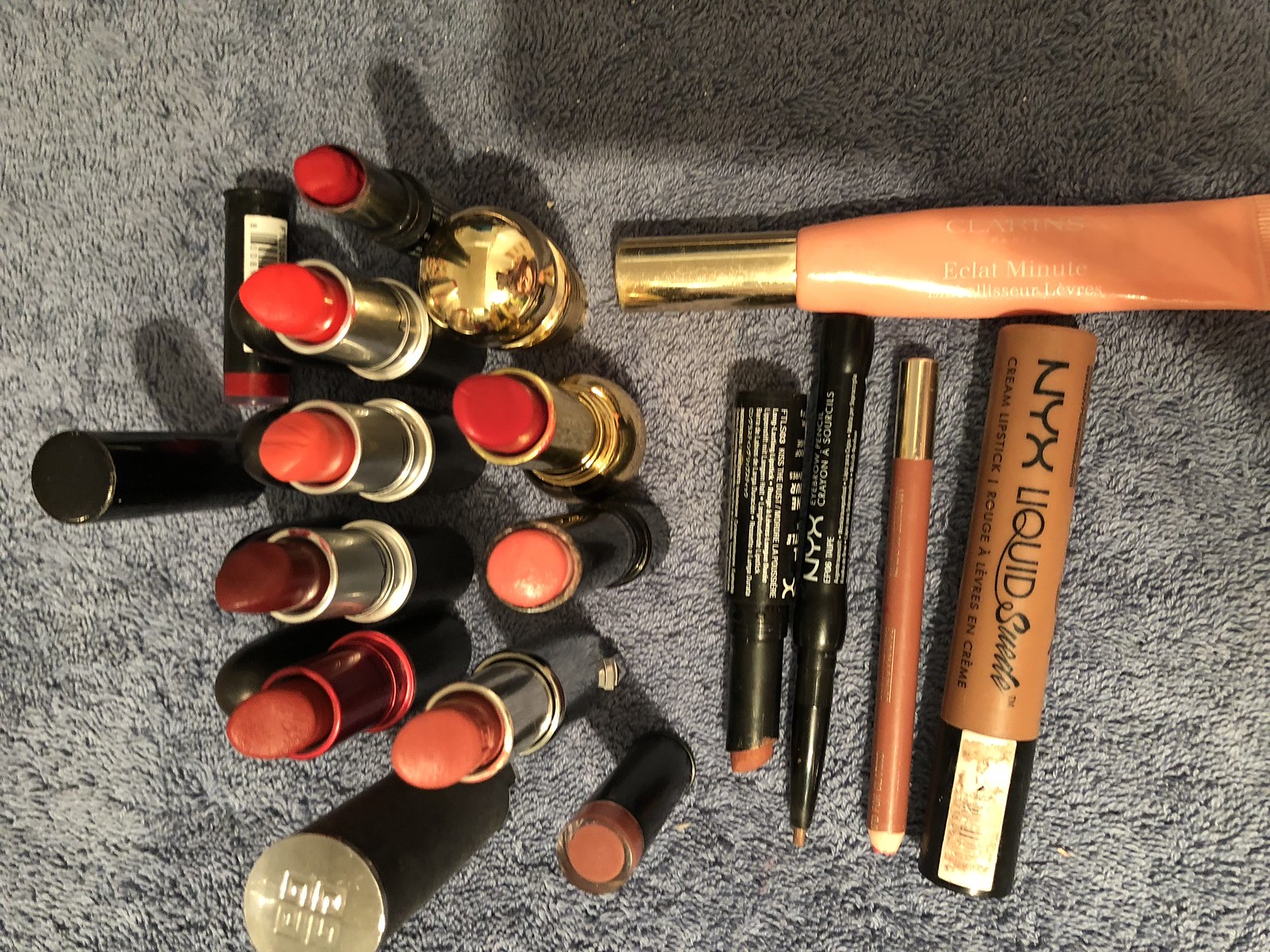The image shows an array of various makeup products meticulously arranged on a plush gray carpet, each casting distinct shadows. At the top, a red lipstick encased in a black container stands prominently. To its right is a gold lipstick container with a shiny red lipstick, featuring a black base. Adjacent to it, a black container with a gold top holds a peachy-orange lipstick.

Next in line is a black-bottomed, gold-topped tube containing brown lipstick. Following this, two containers share a unique design: black bases outlined in red with matching flesh-toned, peachy lipsticks. Nearby, a sleek silver holder also contains a flesh-tone peachy lipstick.

A small closed tube in black is visible, displaying the lipstick color at its top border, and featuring a central circle of matching flesh tone. Behind these, to the left, lies a burgundy lipstick tube horizontal on the carpet, identifiable by a white label with UPC bars and a black tube standing upright beside it.

Additionally, at the bottom left, a gold tube of lipstick stands upright. To its right is a peach-colored tube with a gold cap, inscribed in French. Below that, a skin tone liquid labeled "NYX" and "suede" in black lettering is noticeable, wrapped in a black label with an unreadable white sticker. 

Further to the right lies a flesh-coloured pencil with a gold cap in need of sharpening. A black pen-like stick, possibly an eyeliner, bears the NYX brand. Another black tube, densely inscribed with small white writing, contains flesh-toned lipstick.

The scene is cloaked in intricate shadows from the makeup items, and an indistinguishable shadow hovers at the top of the image.